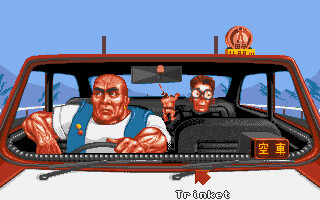This cartoon image depicts a cab driver in an Asian country, as indicated by the Asian script on the back of the meter. The driver is positioned on the right side of the vehicle, which differs from the left-side driver configuration in the United States, adding to the cultural context. The taxi is a vibrant red color, with "TR Inkett" written on it and an arrow that seems to point towards the windshield wiper. Inside the taxi, the driver is accompanied by a passenger who is holding either a drink with a straw or a lit cigarette. The car features two poles extending from its roof, as well as a medallion with red lettering on a yellow background. They are driving through a landscape adorned with mountains in the distance.